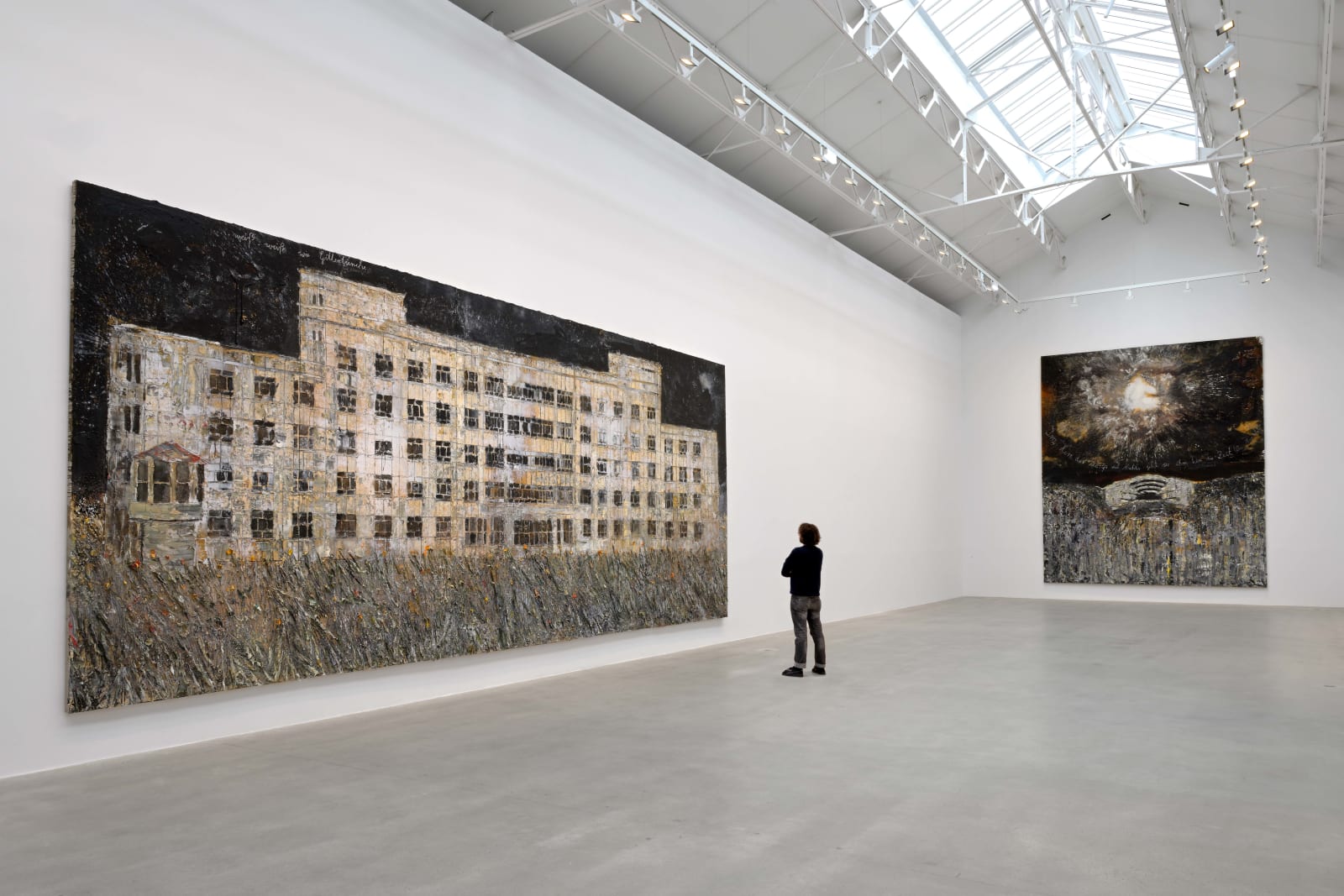In this image of an expansive, white-walled art gallery with a tall ceiling reminiscent of a warehouse, one person, possibly a man, stands slightly right of center, engrossed in observing a large painting. The floor is a sleek, unembellished gray, and the ceiling features an array of spotlights and large skylights with metal rafters. Dominating much of the left wall is an oversized rectangular painting, approximately two and a half to three times wider than it is tall, depicting a large, somewhat monochromatic building with numerous windows, possibly a factory or hospital, set before a stretch of dried, grayish-brown grass. To the man's right, on another wall, hangs a large square painting, its details harder to discern but potentially portraying a bridge and a moonlit scene, slightly obscured by either glare or artistic elements. The room is otherwise empty, accentuating the scale and significance of the artwork.